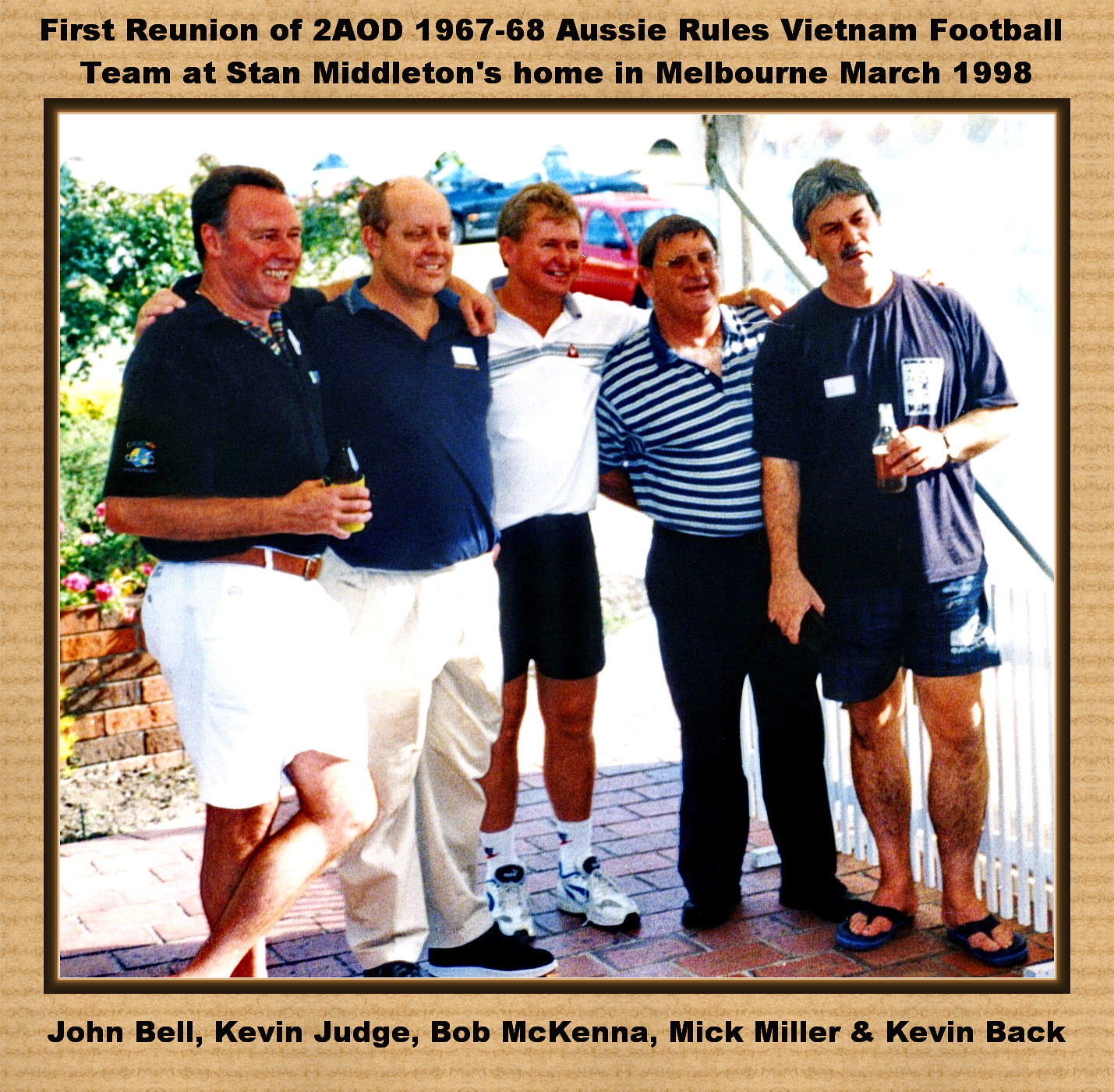In this vibrant image, five middle-aged men, likely in their late 40s or mid-50s, are captured outdoors, standing on red brick pavement. They appear at ease and joyous, with their arms affectionately around each other. All are attired in casual blue and white clothing, with one sporting black pants, and many holding drinks, enhancing the camaraderie of the moment. 

The backdrop is bright and daytime-lit, featuring green bushes and possibly some cars, adding context to their outdoor setting. Above the photograph, elegant black letters announce: "First reunion of 2 AOD, 1967-68 Aussie Rules Vietnam Football Team at Stan Middleton's home in Melbourne, March 1998." Below, the names of the cheerful men are listed: John Bell, Kevin Judge, Bob McKenna, Mick Miller, and Kevin Beck. The photograph is centrally positioned within a light brown square border, framing this moment of reunion and friendship evocatively.